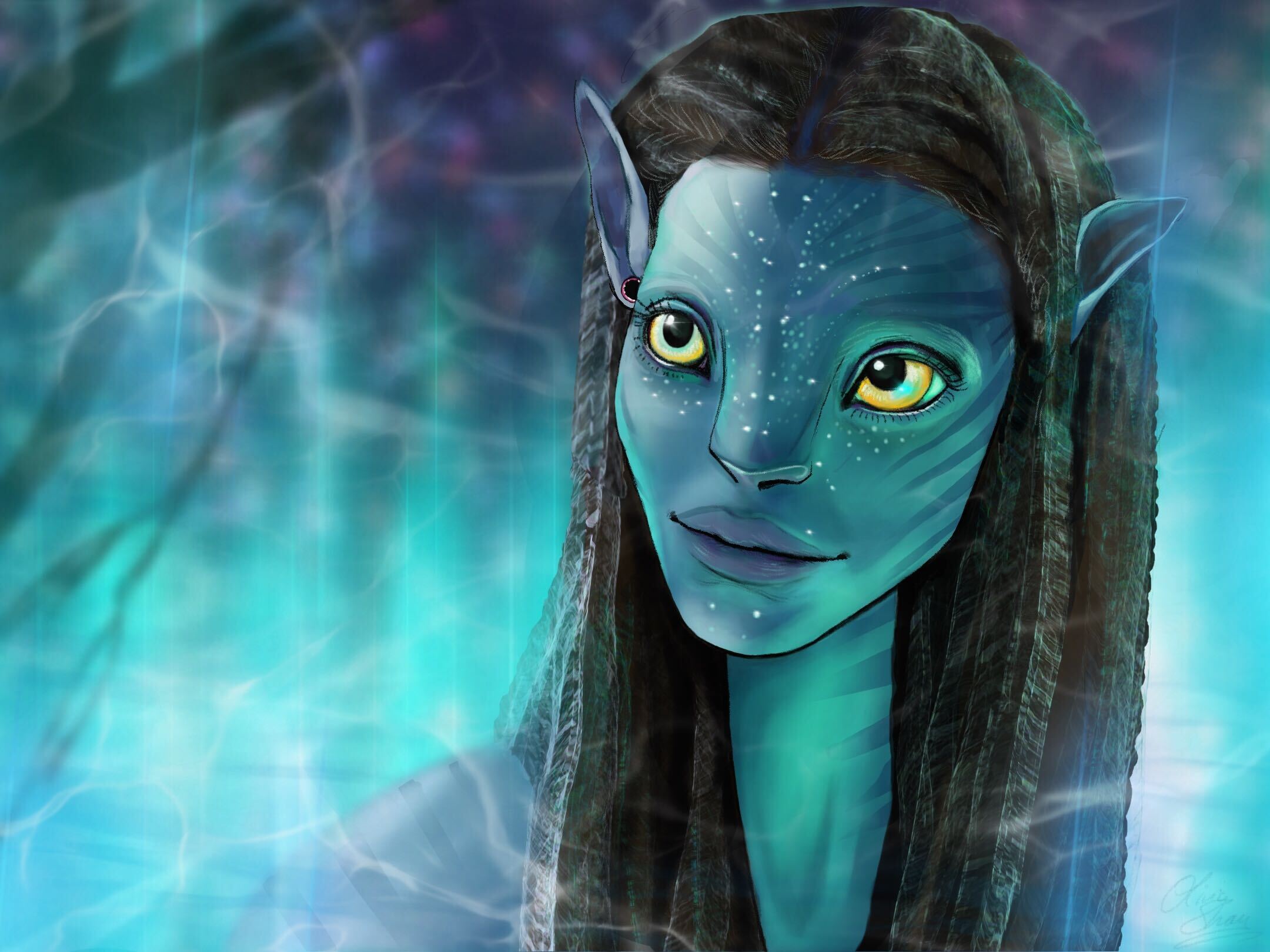This is a highly detailed, artistic rendition of a Na'vi character from the movie Avatar, created in a watercolor style. The character, a female, occupies the right side of the image, gazing contemplatively off to the viewer's left. Her skin is a solid blue, adorned with darker blue tiger-like stripes on her face and neck, as well as white speckles. She has distinct Na'vi features, including large, elfin ears, a broad nose reminiscent of a lion's, cat-like facial features, and striking yellow eyes. Her full lips are a darker blue hue. She has long, black hair styled in dreadlock or braided cornrows that flow from the top to the bottom of the image. The background is a mesmerizing blend of teal, blue, purple, and green hues, reminiscent of light filtering through water or the aurora borealis, with small rays of light accentuating the mystical atmosphere.